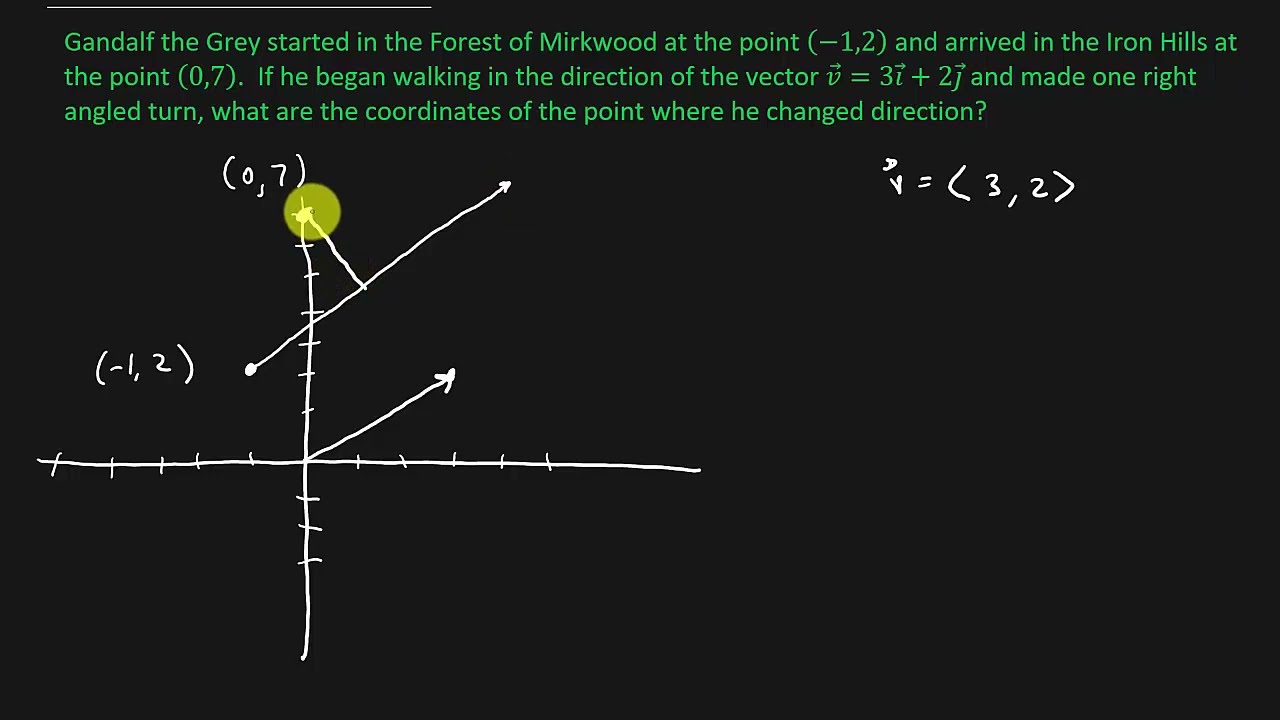The image is an educational graphic reminiscent of what one might find on Khan Academy, featuring an entirely black background. Centered at the top in green text, it reads: "Gandalf the Grey started in the forest of Mirkwood at the point (-1, 2) and arrived in the Iron Hills at the point (0, 7). If he began walking in the direction of the vector v = 3i + 2j and made one right-angled turn, what are the coordinates of the point where he changed direction?" Below this text is a detailed mathematical diagram. On the left side of the image, a coordinate system with two-dimensional axes is drawn in white, featuring dashed lines to denote specific points. The points (-1, 2) and (0, 7) are clearly marked in white chalk. The diagram includes two intersecting arrows: one starting at (-1, 2) and extending upwards to the right, suggesting movement according to vector v = (3, 2), and another starting from the intersection of the axes, also extending to the upper right, indicating the change in direction. To the right of the graphic and beneath the text, a handwritten note shows the variable v within brackets, denoting it as a vector (v = [3, 2]). This comprehensive visual explains a vector-based word problem involving Gandalf's journey and change in direction.